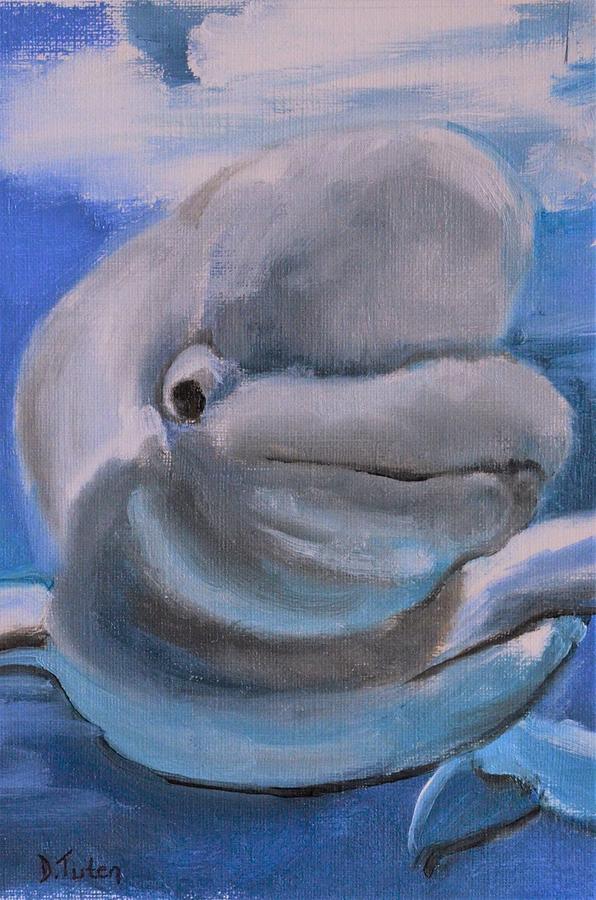This artwork, painted on canvas with what appears to be acrylic paint, showcases a detailed depiction of a grey cetacean, likely a beluga whale, based on its distinctively large, bulbous head and wide mouth. The whale, occupying a central position in the composition, is oriented towards the right side of the frame, with notably white pupils and a black eye that adds an expressive touch to its gaze. The background beautifully transitions from a blue sky adorned with large, puffy white clouds to a darker blue that likely suggests water below, creating a serene aquatic setting. Intricate details, such as potential flippers extending out of the frame and a hint of another whale in the background, add depth to the scene. The piece is signed "D.Tisten" in black on the bottom left corner, affirming its artistic authenticity.